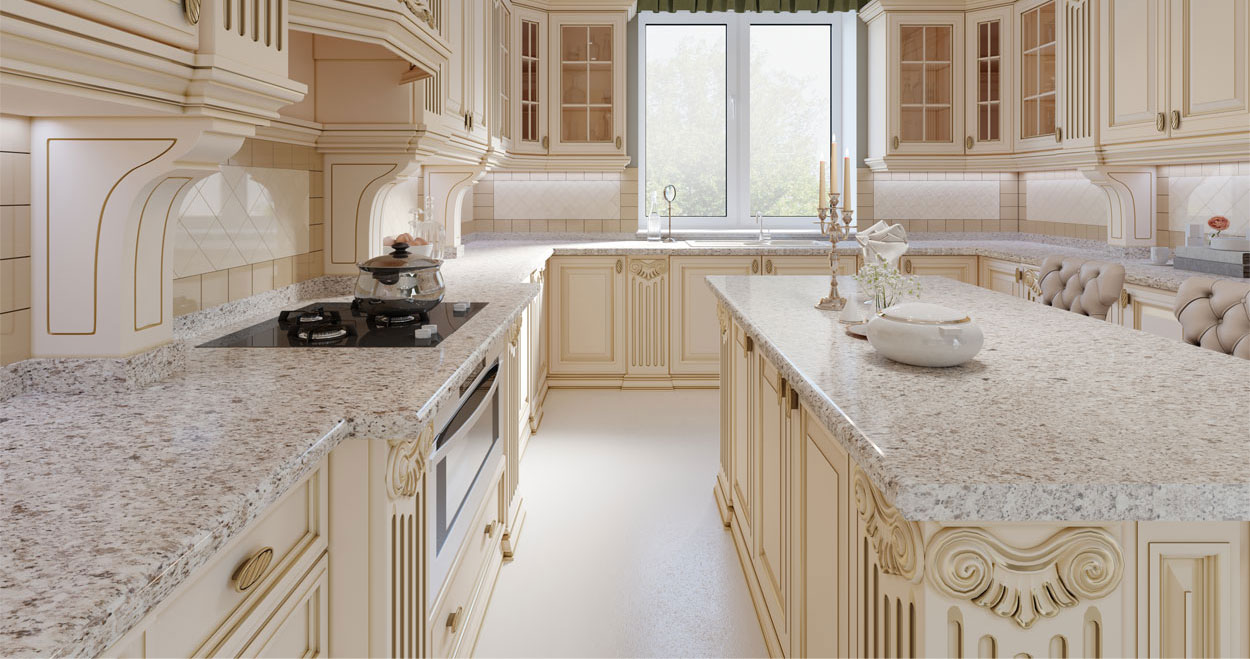This image depicts a spacious, elegant kitchen dominated by a palette of creamy beige and white, with intricate royal-like details. The U-shaped layout features numerous white wooden cabinets and shelves, adorned with delicate Victorian-style embellishments and some glass-fronted doors with small panes. A prominent island stands at the forefront, boasting a sophisticated gray and white marble countertop. On the island, a lit three-candle candelabra, a small vase with white flowers, and a piece of delicate white china add touches of grace and charm. The island is flanked by two padded chairs in a darker beige tone. At the back of the kitchen, a black flat-top stove with an oven beneath is nestled among more marble-topped counters. A large two-way window allows natural light to flood the space, providing a view of the backyard trees. The overall atmosphere is one of modern simplicity, yet the intricate details evoke a sense of timeless elegance. Scattered throughout the kitchen are a few functional items, including plates, candles, and a pot on the stove, maintaining a clean and uncluttered appearance.